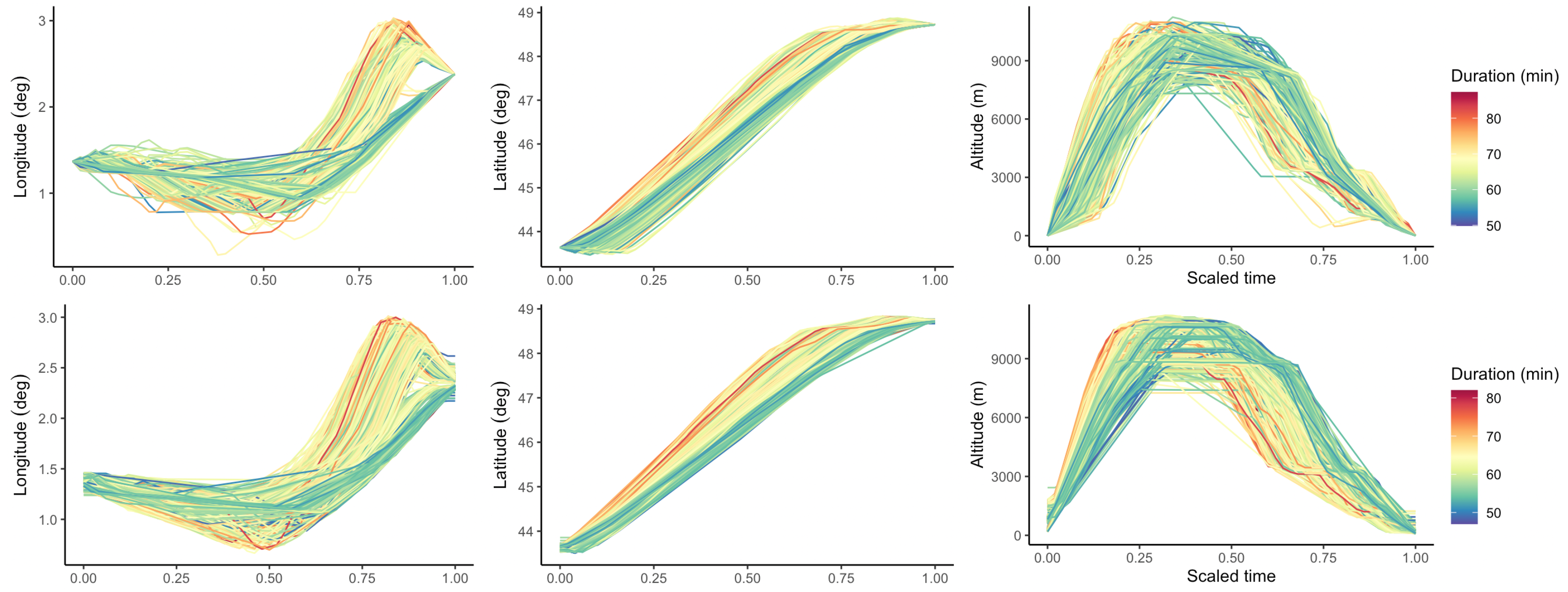In this image, there are six detailed line graphs, each with specific labeled axes. The graphs predominantly feature colors ranging from green to yellow, indicating a sort of duration with the color scale: lower durations are blue, transitioning through green to yellow, with high durations in orange and red. The first and second graphs have axes labeled "longitude" in degrees. The third graph features "altitude" measured in meters on one of its axes, and "scaled time" on the other. Additional details include axes with labels and numbers: Longitude has numbers 1, 2, and 3, while latitude ranges from 44 to 49. The x-axis is demarcated with values at 0, 0.25, 0.5, 0.75, and 1. These annotated features provide a comprehensive look at the various metrics represented, making the graphs informative and visually detailed.